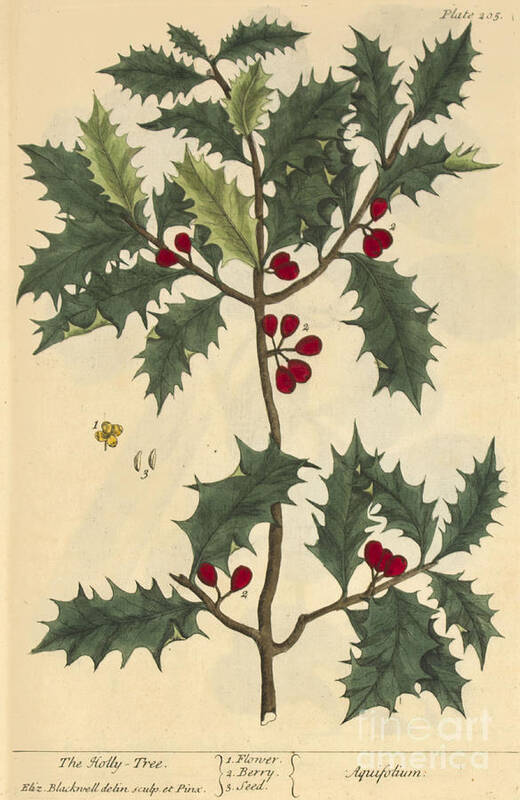The image is a detailed painting of a holly tree, prominently featuring a large, brown and green stem at its center, with four branches extending from it, two on each side. These branches are adorned with numerous wide, long leaves that vary in shades of dark and light green. Interspersed among the leaves are several red berries, giving the plant a vibrant appearance. Additionally, there are flowers visible, with one yellow flower specifically noted on the left side, near which two seed-like structures resembling rice grains can be observed. The background is light peach, creating a subtle contrast with the vivid colors of the plant. Written in black text at the top right corner of the painting is "Plate 205," and below the plant’s depiction, more textual information is provided, identifying the holly tree and labeling different parts of the plant, including numbered annotations for a flower, berry, and seed.